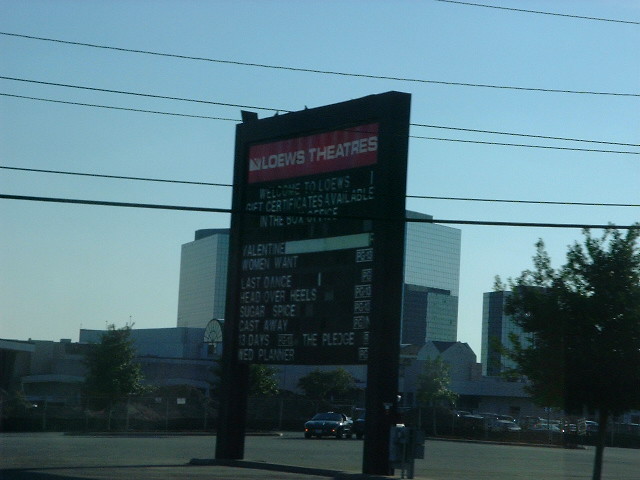The color photograph captures an outdoor scene featuring a bustling parking lot lined with numerous cars and flanked by commercial buildings. Dominating the foreground, a large black sign with bold white lettering and a prominent red rectangle reads "L-O-E-W-S Theatres." The red rectangle accentuates the Lowe's branding, while additional sections in black with white text announce various movie showings, including "Valentine," "What Women Want," "Last Dance," "Head Over Heels," "Sugar & Spice," "Cast Away," "13 Days," "The Pledge," and "The Wedding Planner," each accompanied by their respective showtimes. A small, dark green tree is visible to the right of the image. Stretching across the scene, a network of black electrical and phone lines adds to the urban feel. The sky above is a clear blue with soft white cloud accents, providing a scenic backdrop to the busy environment.